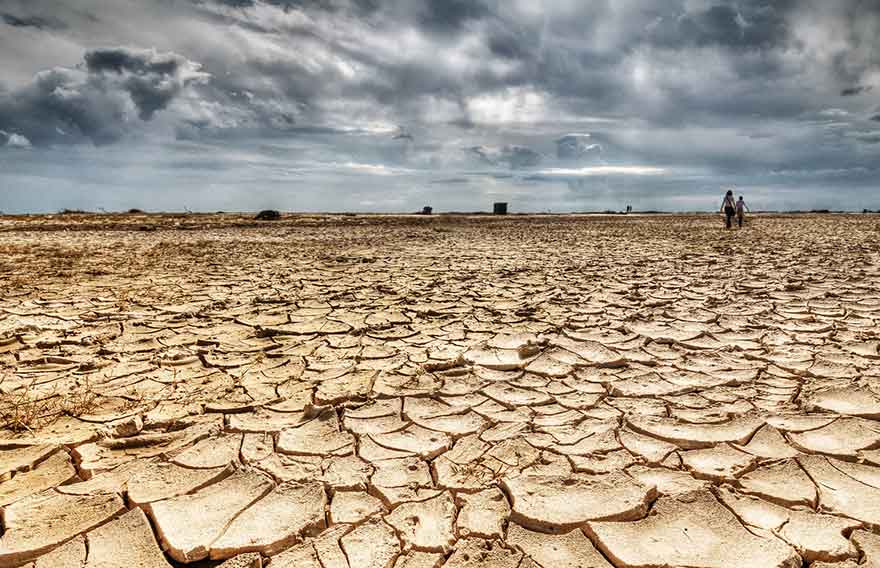The photograph captures an expansive, barren desert or salt flat that stretches across the frame, roughly twice as wide as it is tall. Dominating the bottom two-thirds of the image is a cracked, arid landscape, characterized by tan-colored earth split into an intricate pattern of triangular and geometric shapes. This desolate ground, devoid of any sign of moisture, suggests a region that seldom experiences rain.

In the upper third of the image, an overcast sky looms menacingly, filled with turbulent gray clouds that blanket the scene, adding to the austere atmosphere. Despite the menagerie of gray tones that suggest a storm might be brewing, the parched land below contradicts this impression, reinforcing the arid nature of the environment.

On the right side, near the center-top portion of the image, two small figures—a man and a woman—can be seen walking away from the camera towards the horizon. Their presence adds a sense of scale to the vast emptiness surrounding them. Additionally, there are indistinct dark blobs scattered in the distance, their details lost in the flat light of the scene, further emphasizing the stark and remote setting. The photograph’s color palette is dominated by muted tones of white, gray, blue, tan, black, and brown, depicting a harsh, outdoor environment.